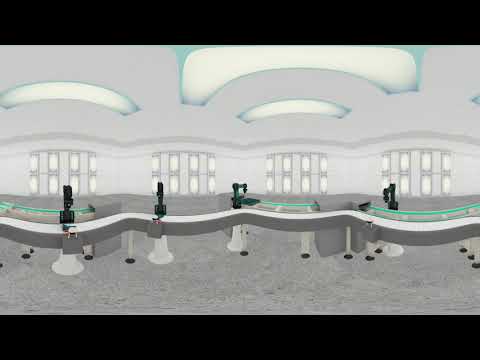In a digitally rendered, somewhat pixelated image that appears to be a panoramic view likely designed for augmented or virtual reality, we observe a meticulously detailed gray room. Dominating the foreground, a sinuous gray line resembling an assembly line weaves back and forth like a snake across the gray carpeted floor. Running parallel above it is a white, curved countertop supported by slender white stands. This countertop appears to hold black, statuesque items with overhanging structures that evocatively resemble sewing machines or perhaps sink fixtures, but their exact function remains ambiguous due to the image's low resolution.

The background features a distinct architectural setup with four sets of arched walls, each adorned with eight white-framed windows outlined gray, contributing to the room's well-lit ambiance. Additionally, the light gray ceiling is punctuated by light fixtures with centers of white light, radiating a teal fade around them. Despite several interpretations ranging from a potential bathroom or waiting area to a museum ramp, the exact nature and purpose of the room remain enigmatic, exacerbated by the image's blurred quality. Overall, the scene is characterized by an abundance of gray tones and an airy, expansive feel devoid of any human presence.